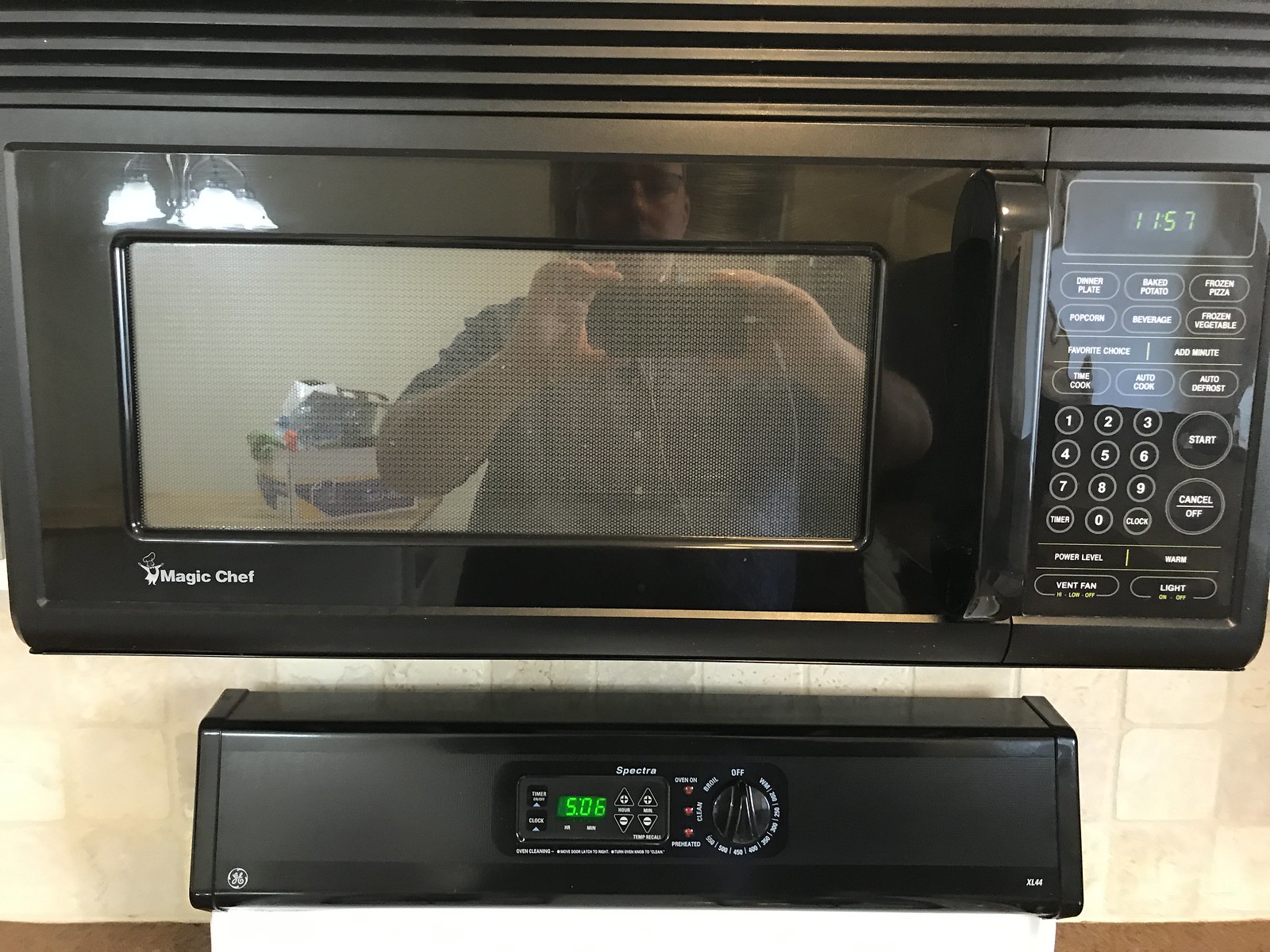This detailed color photograph captures a narrow GE stove with a black Magic Chef microwave mounted above it. The microwave, positioned where an exhaust hood would typically be, features a shiny, touch-button panel and a digital display showing the time as 11:57. A reflection of the person taking the photo, holding a smartphone horizontally, is clearly visible on both the microwave’s glossy surface and its glass door. The individual appears to be a Caucasian woman, and the background reflection includes a tea cart or wine rack and pendant ceiling lights with glass ruffle shades. Additionally, the wall behind the microwave and stove showcases a backsplash of light beige, earth-toned square tiles. The stove’s display indicates a setting for 506, presumably how much time remains for something currently being cooked in the oven. The stove is branded with white lettering that reads "Spectra."